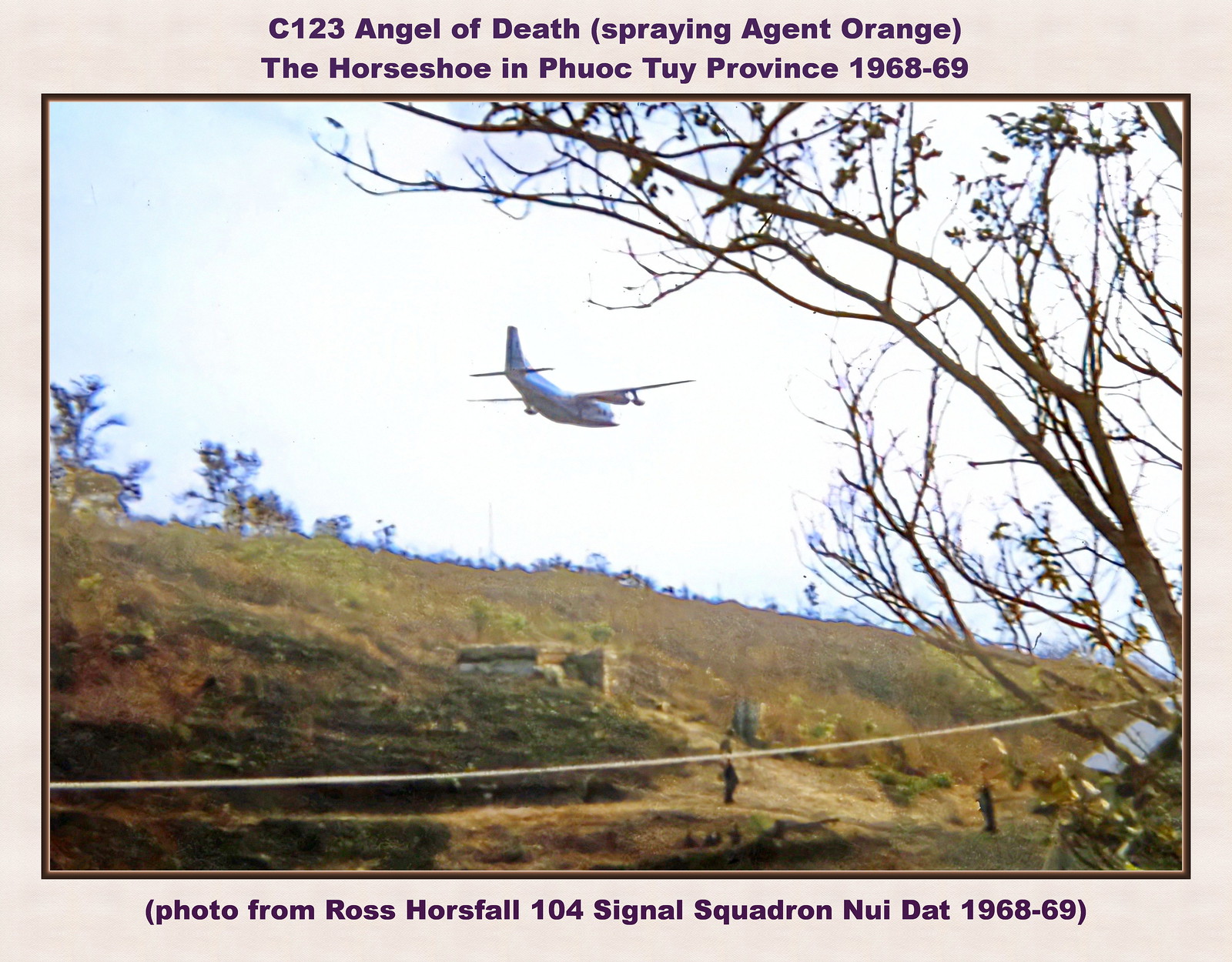This photograph, taken during the Vietnam War in 1968-69, depicts a C-123 airplane, dubbed the "Angel of Death," flying low over a hill in Phuoc Tuy Province. The aircraft was likely involved in spraying Agent Orange, a defoliant used during the war. The distant shot captures the plane moving through a clear, bright blue sky, above a landscape characterized by beige and green hues, indicating sparse vegetation and a hill with scattered foliage. A slender tree, with few leaves, rises from the right side of the frame, stretching upwards. The image is bordered in beige-gray, with a caption at the top reading "C-123 Angel of Death, Spring Agent Orange, The Horseshoe, Phuoc Tuy Province 1968-69" and a bottom note stating "Photo from Ross Horse Fall, 104 Signal Squadron, Nui Dat 1968-69."